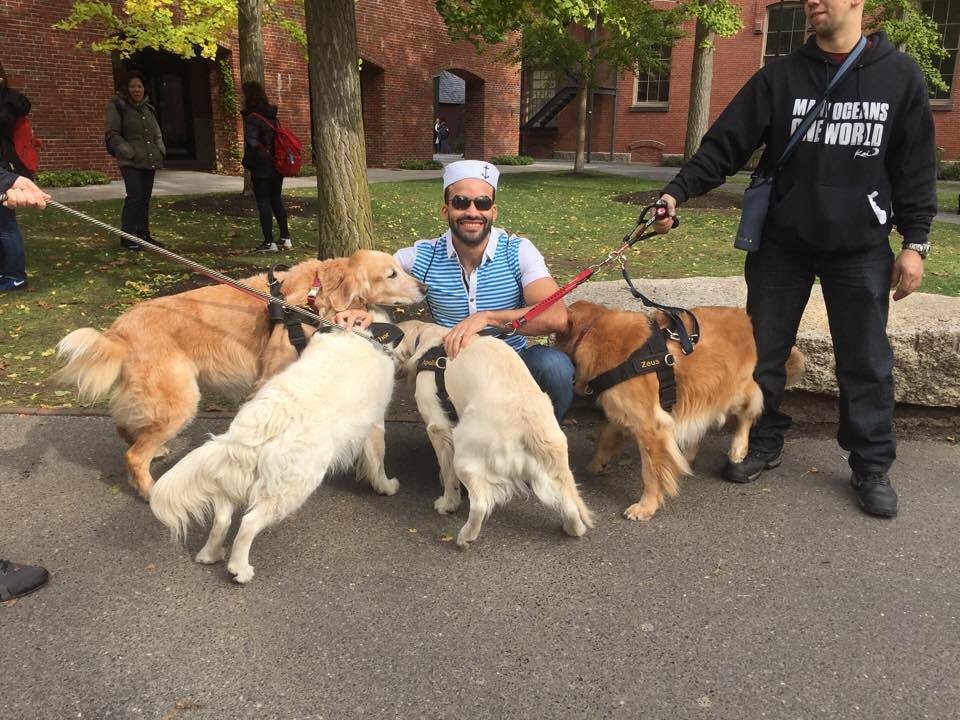In this detailed photograph set against the backdrop of reddish brick buildings and a small patch of grass with green-leaved trees, a young man is the focal point, squatting down on a city sidewalk surrounded by four affectionate golden retrievers. The buildings in the background display beautiful archways, large windows, and steps, suggesting a public courtyard area, possibly on a college campus. The young man, sporting sunglasses, a closely shaved beard and mustache, is joyfully smiling at the camera. He wears blue jeans, a blue and navy striped shirt, and a white hat adorned with an anchor, giving it a sailor-like appearance. The golden retrievers, two of a darker golden hue and two lighter, form a semi-circle around him, each vying for his attention. To the right, a man dressed entirely in black, with a hoodie featuring the phrase "Make oceans one world," holds a red leash connected to one of the dogs. In the backdrop, three women engage in conversation, adding a touch of everyday life to the scene. This photograph captures a tender moment of connection and joy amidst a vibrant community setting.